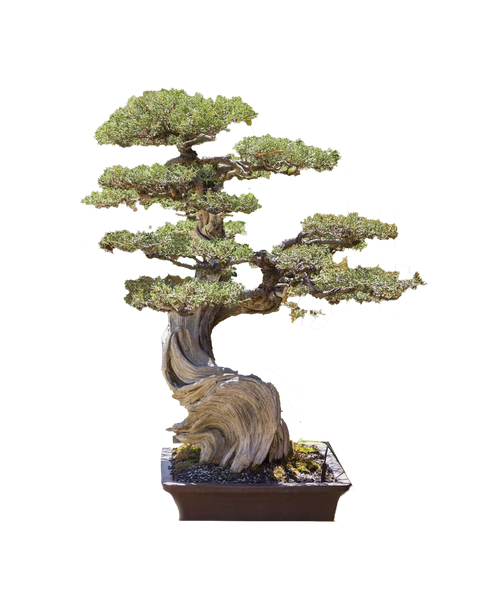The image shows a detailed, color photograph of a bonsai tree positioned in a shallow, square, brown planter with a base of black gravel and soil. The bonsai's trunk is disproportionately thick and intricately gnarled, suggesting age and resilience, with a textured, aged appearance that alternates between brown and grayish tones. Its twisted limbs extend horizontally, forming distinct, flat, platform-like arrangements of fine green leaves that resemble cloud layers. These platforms create a multi-level structure, with four main tiers of leafy branches, each exhibiting wave-like contours. The sunlight illuminates the scene, casting light on the bonsai and highlighting the planter's details and the intricate texture of the trunk and foliage.